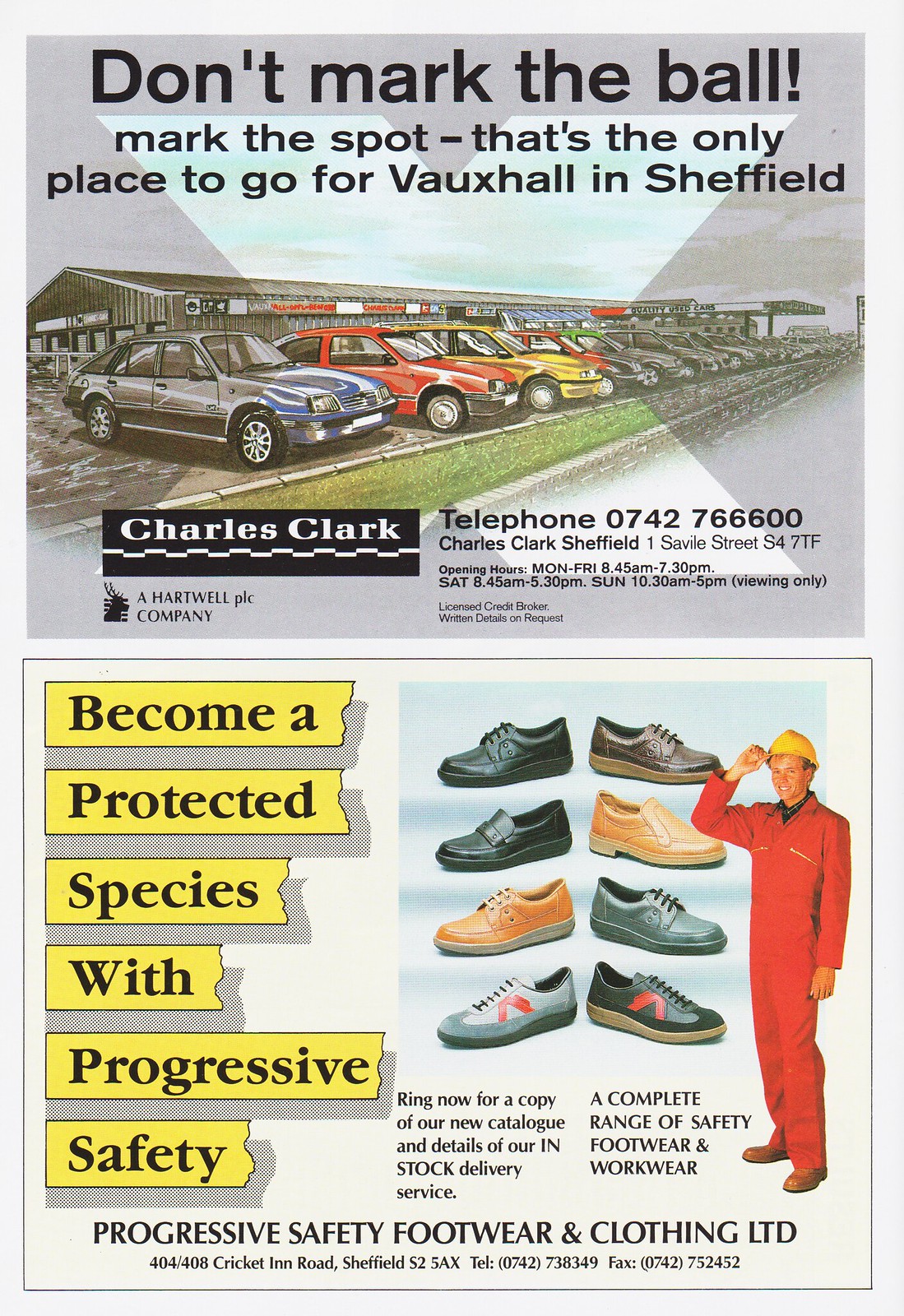This vertical rectangular image, likely from an advertisement page in a sporting event program, is split into two distinct sections. The upper section advertises Charles Clark, a car dealership in Sheffield specializing in Vauxhall vehicles. Dominating this section is the bold black text, "Don't mark the ball! Mark the spot." This slogan is followed by the declaration, "That's the only place to go for Vauxhall in Sheffield." Beneath the text lies an image of neatly rowed automobiles, possibly Vauxhall models, resting on asphalt with a grassy curve detail on the edge. The dealership's branding includes a black rectangle with "Charles Clark" in white letters to the left, and detailed contact information on the right. This includes a phone number, address at 177 Savile Street, Sheffield S4 7UQ, and their operating hours: Monday to Friday, 8:45 AM to 7:30 PM, Saturday until 5:30 PM, and Sundays from 10:30 AM to 5 PM. Additionally, it mentions the dealership is part of Hartwell Company PLC and is a licensed credit broker.

The lower section promotes progressive safety footwear, featuring a man in a red jumpsuit and yellow hard hat. The advertisement's background is gray with bold text in yellow rectangles stating, "Become a protected species with progressive safety." To the right of this figure is an array of safety shoes in various colors and designs. Below this, it advises to "ring now for a copy of our new catalog and details of our in-stock and delivery service." Further text highlights the "complete range of safety footwear and workwear" provided by Progressive Safety Footwear and Clothing Limited. Contact information for this company includes a Sheffield address at 404/408 Cricket Inn Road, S5 AX, a telephone number 0742 738 349, and a fax number 0742 752 074.